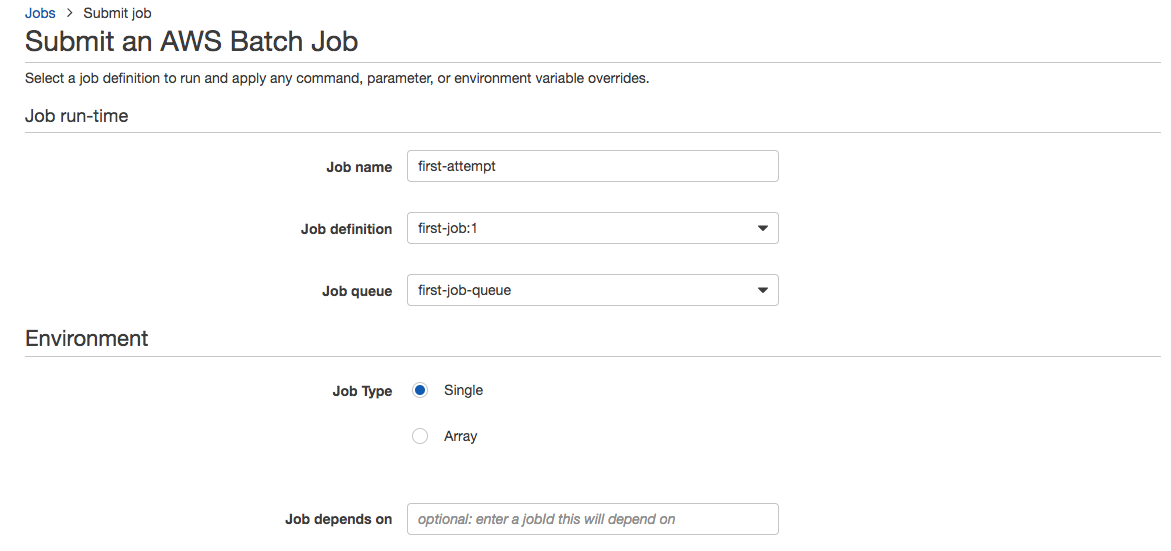Screenshot of AWS Console Submission Page for Batch Job

At the top of the screenshot, there is a section labeled "Jobs" with an option to "Submit Job" directly below it. The highlighted section is titled "Submit an AWS Batch Job." This section guides users to select a job definition to run and apply any command parameters or environment variable overrides.

Below this guidance text, there is a section titled "Job Runtime," which includes three input fields:

1. **Job Name:** The top input field is labeled "First Attempt," where users can type in the name of their job.
   
2. **Job Definition:** This is a drop-down menu, currently showing "first job:1." Users can select from previously defined job definitions.

3. **Job Queue:** This drop-down menu is labeled "First Job Queue," where users can select the job queue their job will be submitted to.

The final section, labeled "Environment," includes several parameters:

- **Job Type:** Users can select between "Single" or "Array" job types, allowing for either individual or multiple job submissions.
  
- **Job Depends On:** This optional field allows users to enter a job ID that their current job will depend on, specifying a job dependency.

This detailed step-by-step interface helps users configure and submit batch jobs efficiently on the AWS platform.